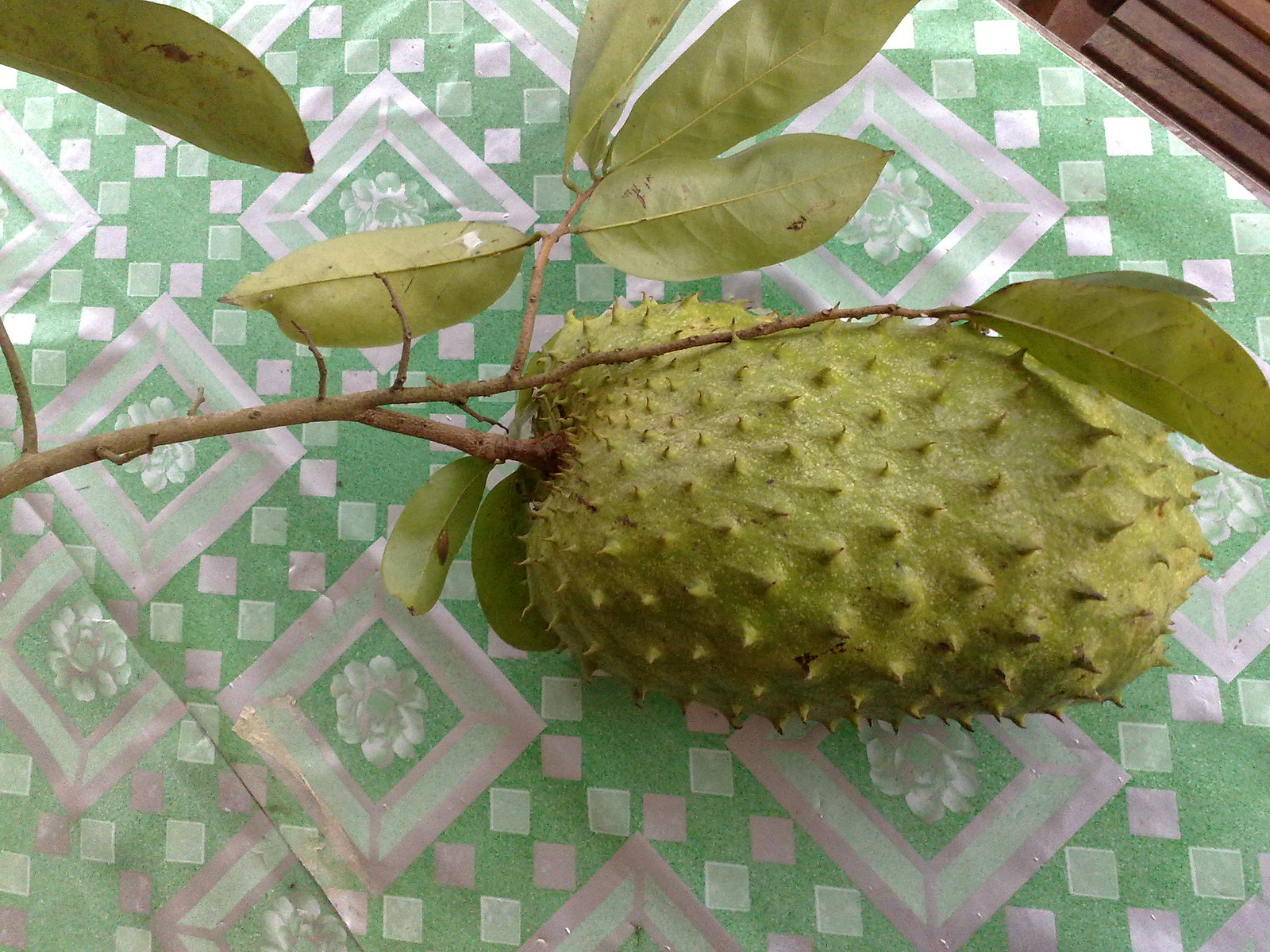This is an image of a unique, spiked green fruit with an elongated oval shape, still attached to its cut-off tree stem. The stem features eight visible leaves, which are light green with some brown, dying spots. The fruit and stem rest on what appears to be a wooden bench covered with a tablecloth. The tablecloth has an intricate pattern comprised of squares and diamonds, each containing a flower with white and pink petals. The background is a combination of green, purple, and white, featuring repetitive diamond designs each enclosing similar flower patterns. The lighting is diffused, suggesting it was taken under overcast skies, creating a soft shadow effect.